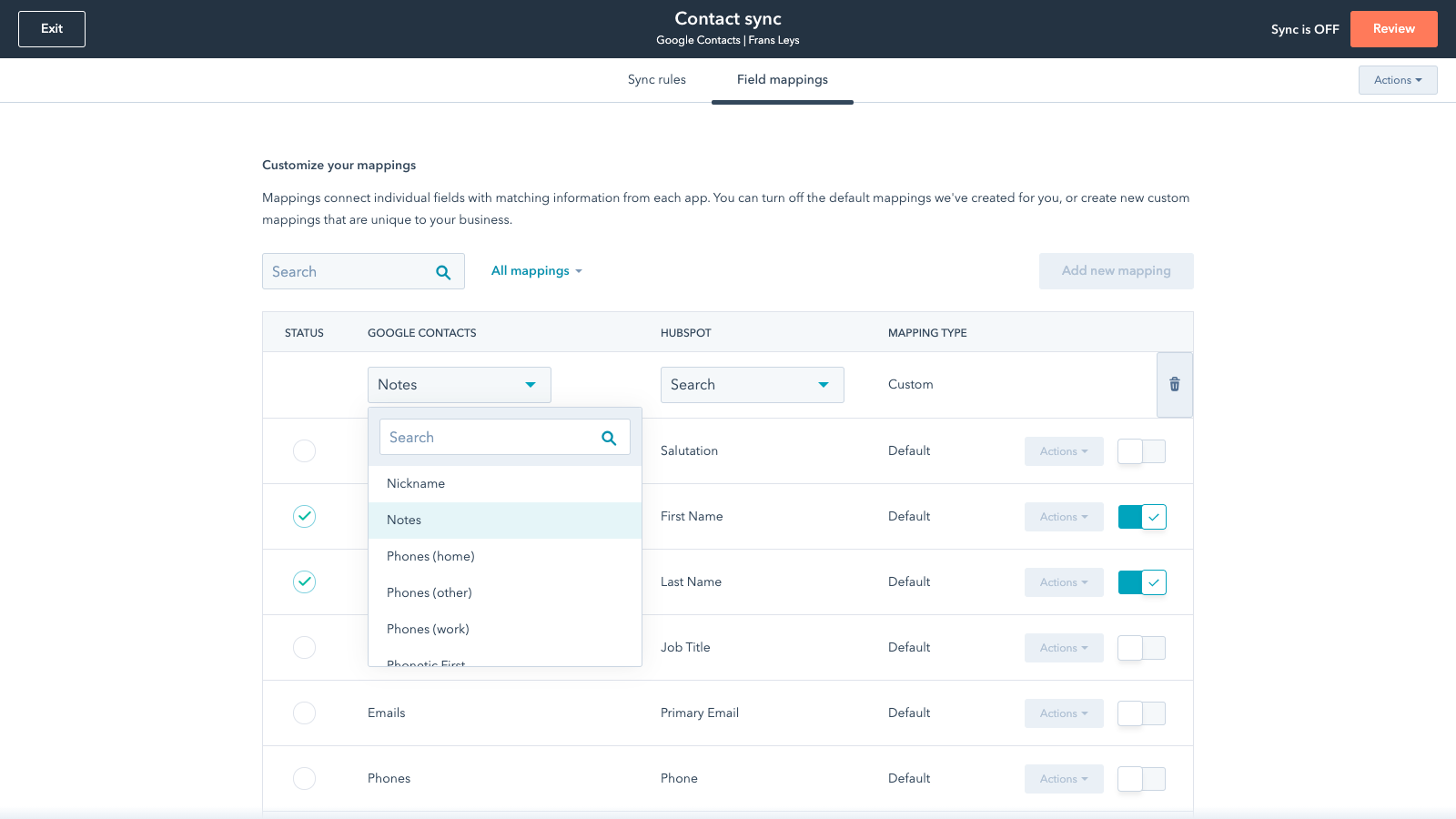The image is a screenshot of a web page designed for managing contact synchronization. The page is displayed in a horizontal, landscape orientation within a rectangular frame. The overall background of the page is white, but it features a prominent black border running along the top, which serves as a header.

In this black header, a few important buttons and text elements are visible. On the left side, there's an "Exit" button, and on the right, a red "Review" button, next to which the text "Sync is off" is displayed. Centrally located in this header is the title "Contact Sync" in large font, accompanied by "Google Contacts / Friends Keys" in a slightly smaller font beneath it.

Below this header, in the white portion of the page, is a centered section with two tabs labeled "Sync Rules" and "Field Mapping," the latter of which is underlined to indicate it is currently selected. 

Beneath the "Review" button, there is another button labeled "Actions." The main section of the page, titled "Customize Your Mappings," displays a table with multiple columns, including "Status," "Google Contacts," "HubSpot," and "Mapping Type." Each column features drop-down menus allowing for various customizable options.

Further down the table, specific fields such as "Salutation," "First Name," "Last Name," along with other options like "Emails," "Phones," etc., are listed for detailed contact information mapping. This page appears to be a detailed interface for configuring and managing how contact information is synchronized between platforms.